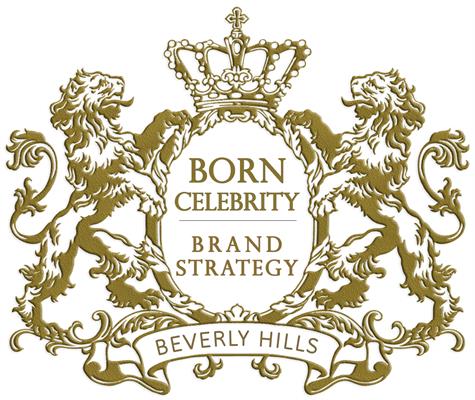The logo is an elaborate, golden design featuring two regal lions standing on their hind legs with tongues sticking out, flanking an ornate oval shape at the center. Each lion has its paw resting on the oval. The oval, resembling an egg or a ring, is crowned with a majestic, jewel-encrusted crown that has a cross at its pinnacle. The interior of the oval bears the inscription "Born Celebrity Brand Strategy." Beneath the main emblem, a decorative ribbon unfurls with the text "Beverly Hills." The entire logo is intricately detailed, exuding a sense of prestige and grandeur reminiscent of traditional coats of arms.